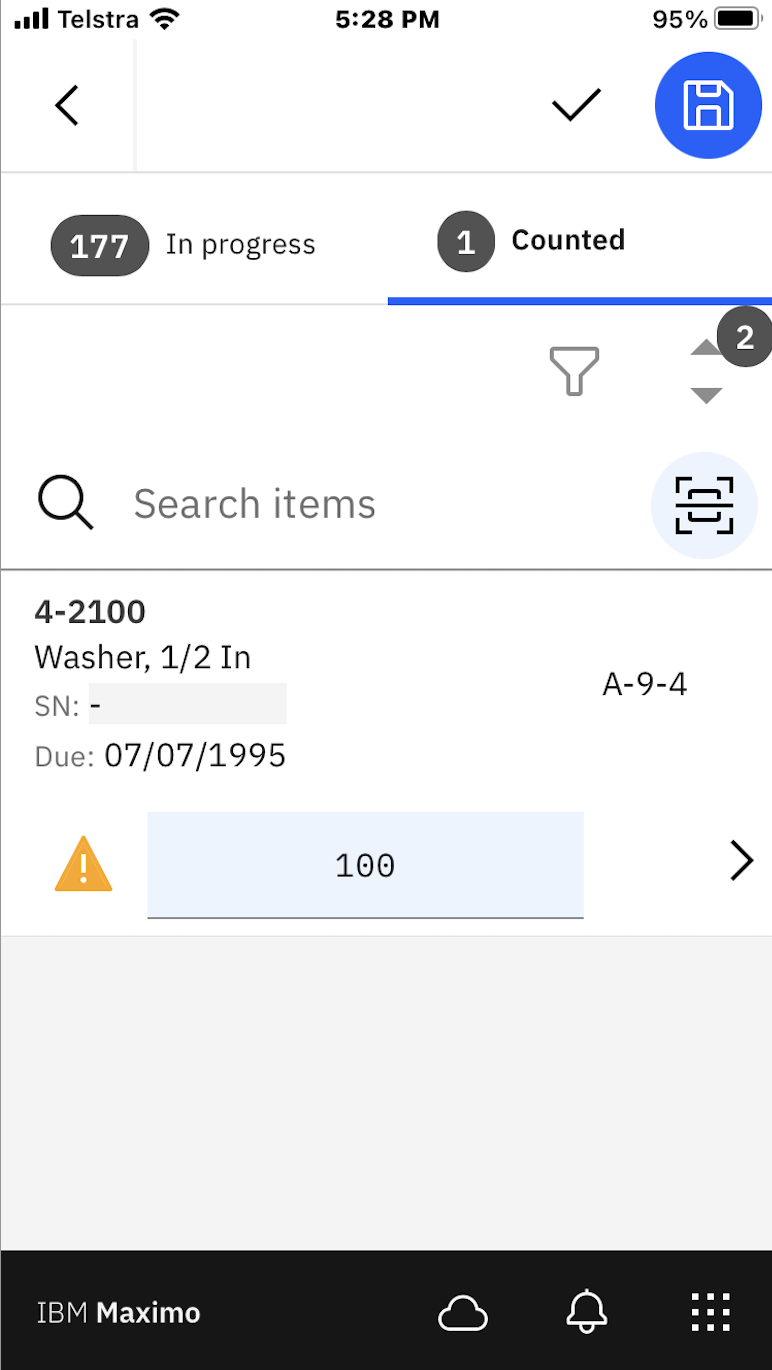This is a detailed screenshot of a website displayed on a mobile phone. The screenshot captures various elements, predominantly from a web application, likely IBM Maximo. 

At the top of the screen, the device status is shown with the battery life at 95%, the time displayed as 5:28 PM, and the Wi-Fi signal indicating the device is connected to a network. The carrier information, Telstra, is visible in the top left corner.

Below the device status bar, there is a header displaying the title "IBM Maximo" accompanied by a bell icon, a cloud icon, and a list icon, suggesting notifications, cloud services, and archived lists respectively.

In the main section of the screenshot:
- There are multiple tabs displayed. One of the tabs is labeled "In-progress" with an indicator showing '177' items, and another tab labeled "Counted" showing just '1' item.
- To the right, an icon resembling a hard disk, colored blue, is visible.
- Beneath these tabs, there is a search bar with a magnifying glass icon, suggesting a search functionality.

Further down, there are labels and fields including:
- A label "4-2100" followed by "washer, 1/2 IN."
- A field labeled "S/N" which is currently blank.
- Another field "DO" with the date "7-7-1995".

The overall structure gives an impression of a detailed interface for managing or tracking items, possibly within an inventory or maintenance system.